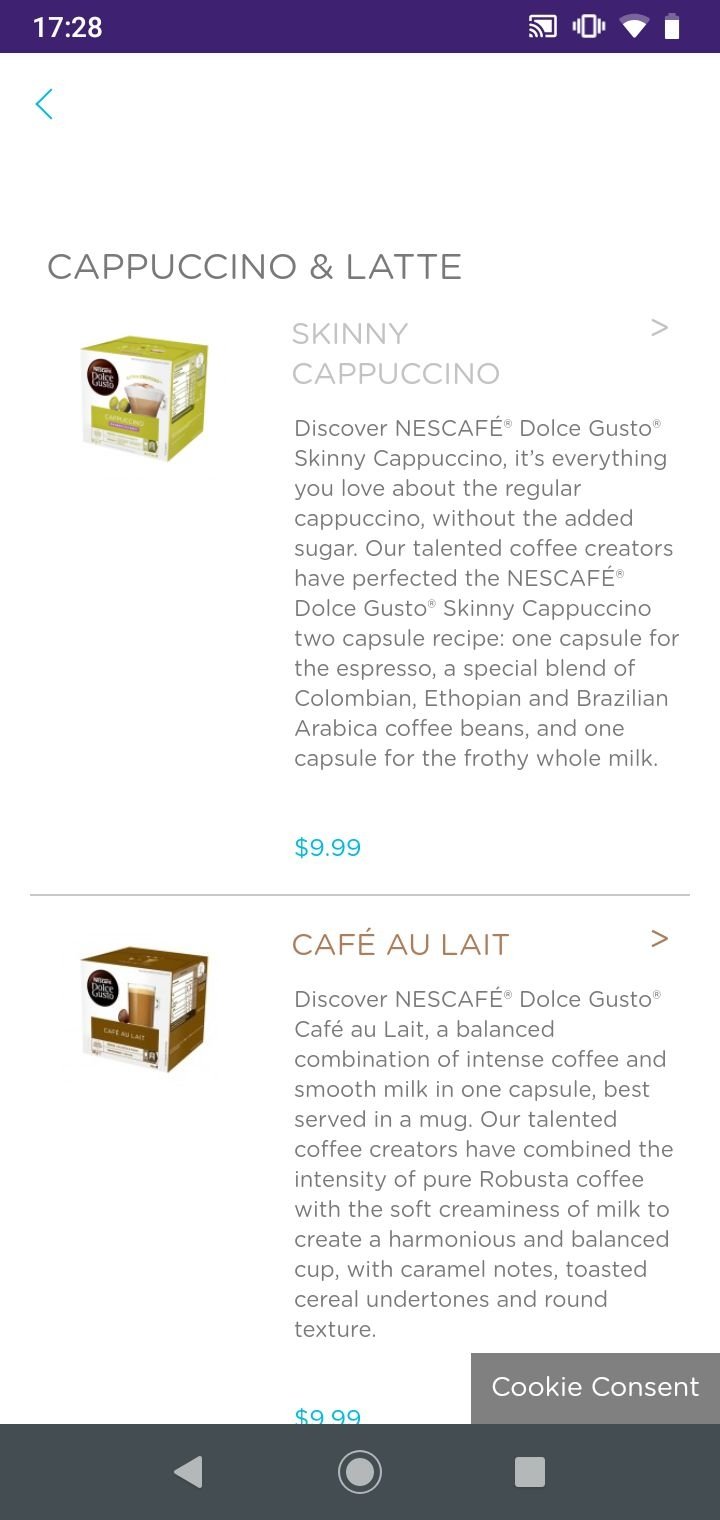This image is a detailed screenshot from a website. At the top, it features a dark purple banner with the text "1728" in white on the left. On the right side of the banner, there are icons for Wi-Fi or cell signal and a battery indicator. Below the banner, a turquoise arrow pointing left is set against a white background.

Underneath, the text "CAPPUCCINO LATTE" is displayed in large, black capital letters. Below this heading, there is a graphic of a product box followed by a description: "Skinny Cappuccino - Discover Nescafe Dolce Gusto. Skinny Cappuccino is everything you love about regular cappuccino without the added sugar. Talented coffee creators have perfected the Nescafe Dolce Gusto Skinny Cappuccino two-capsule recipe: one capsule for the espresso, a special blend of Ethiopian, Colombian, and Brazilian arabica coffee beans, and one capsule for frothy whole milk." The price is listed as $9.99.

Further down, the site introduces another product: "COFFEE A LOT - Discover Nescafe Dolce Gusto. Coffee A Lot is a balanced combination of intense coffee and smooth milk in one capsule, best served in a mug. Talented coffee creators have combined the intensity of pure robust coffee with the soft creaminess of milk to create a harmonious and balanced cup with caramel notes and cereal undertones, featuring a rounded texture." This product also is priced at $9.99.

At the bottom of the image, there is a "Cookie Consent" notification.